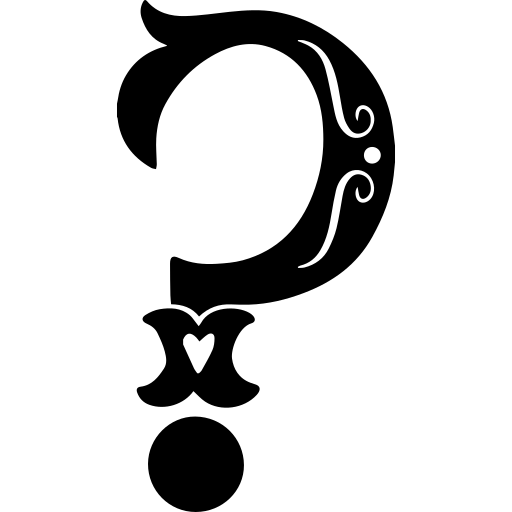The image features a large, ornate question mark composed of three distinct black segments set against a pure white background. The top part of the question mark forms a backwards 'C', adorned with two symmetrical white curly cues and a white dot centered between them, giving it a decorative flourish. Below this, the midsection resembles a stylized, curvy 'X', with its intersecting lines creating a white heart shape in the center. Completing the question mark, a solid black circle rests at the bottom. The entire design appears to float on the white background, without any visible borders or edges, highlighting the bold, black lines and intricate details of the illustration.